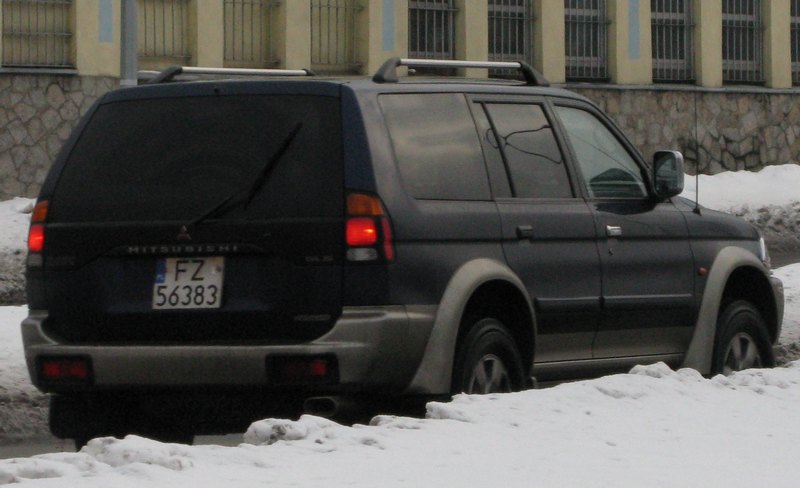In this landscape-oriented photograph, a large black Mitsubishi SUV, with distinctive silvery-gray trim, is the focal point. Parked on a snow-covered street, the vehicle is surrounded by a thick blanket of white snow that reaches up to mid-tire level. The rear of the SUV prominently displays the Mitsubishi name in shiny silver-gray lettering, accompanied by the iconic triangle-shaped Mitsubishi logo. The license plate, marked "FZ 56383" in black lettering, is clearly visible. On the roof of the SUV, a silver and black bike rack is mounted, with one silver pole on each side. 

In the background, a substantial building is partially visible. The lower portion of the structure is constructed of stone, while the upper part appears to be made of concrete. The façade features a pattern of concrete columns and blue stripes, with numerous windows covered by metal bars, suggesting it might be an institutional building. The icy environment captured in the image emphasizes the cold conditions, further highlighted by the slushy snow on the street and the taillights of the SUV, suggesting some movement or recent stopping.